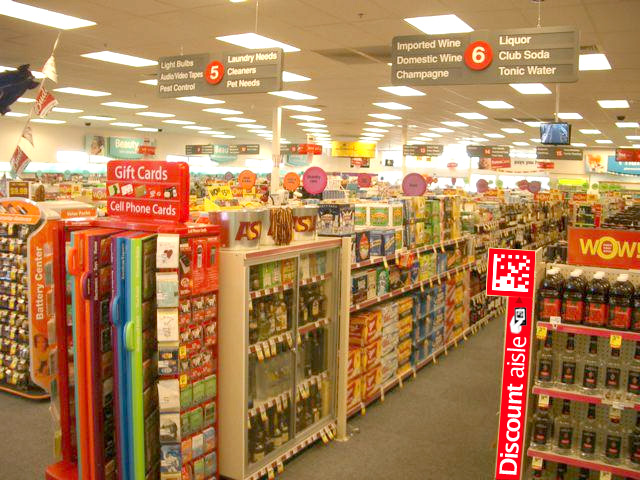This color photograph captures the bustling interior of a well-stocked drugstore, as viewed from a vantage point that looks down several aisles. Prominently displayed, two signs hang from the ceiling, each labeled with different aisle numbers and their respective product categories. 

On the left side, the gray sign with bold, white lettering reads: "Aisle 5," and detailed beneath it are the items available: light bulbs, audio tapes, pest control products, laundry needs, cleaners, and pet necessities. Opposite it, on the right, another suspended gray sign identifies "Aisle 6," listing its own array of products: imported wine, domestic wine, champagne, liquor, club soda, and tonic water. 

The scene is bright with overhead lights illuminating the gray-carpeted floor, adding to the welcoming atmosphere. Positioned on the right side of the image is an additional sign labeled "Discount Aisle," suggesting special deals and promotions available in that section. The photograph captures the orderly and well-signed nature of the store, facilitating easy navigation and an efficient shopping experience for customers.